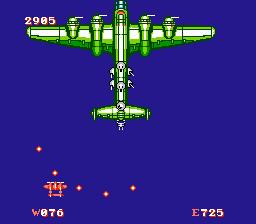This square image appears to be a screenshot from a video game, featuring a dynamic aerial combat scene. Dominating the frame is a green fighter plane, positioned centrally and heading upwards toward the top of the image. The plane, decorated with intricate skull designs on its shorter back wings, showcases a color palette of green, dark green, light green, and white. Its long front wings extend outwards, giving it a sleek and menacing appearance.

In the bottom left of the image, a smaller, distinctly orange and pink plane is captured mid-flight. From this vibrant aircraft, a series of five bright fireballs arc forward, hinting at an ongoing attack or defensive maneuver. The vivid contrast between the two planes creates a sense of urgency and action in the scene.

Additional details include numerical indicators: "2905" is situated just above and to the left of the small plane, while "W076" is written below it. In the bottom right-hand corner of the image, "E725" is prominently displayed. These alphanumeric sequences likely serve as in-game coordinates or scores, adding an extra layer of context to the intense aerial battle depicted.